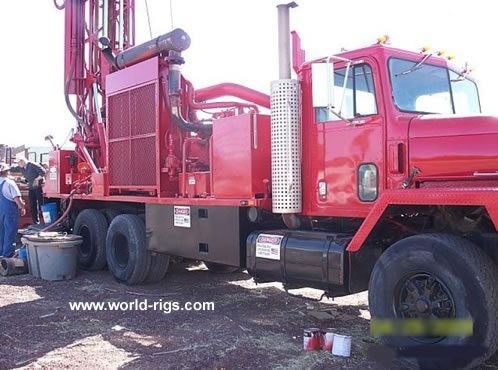The photograph captures a side view of a large, red flatbed truck, occupying most of the image's frame and stretching from the left to the right. The truck is outfitted with several square-like pieces of red-painted equipment on its flatbed, consisting primarily of hydraulics and pumps, connected by various tubes. At the very back, a crane or large pump is visible, supported by silver hydraulic arms. The black rubber tires are fitted with black rims, and black boxes labeled "Danger" are mounted under the truck's cab. In the bottom left corner of the image, white text reads, "www.world-rigs.com." Two men are positioned near the truck; one is wearing blue overalls and a hard hat, while the other wears a light-colored baseball cap and a dark sweater. Three cans are situated next to the front tire. Additionally, there are cans of paint near the back tires. The front end of the truck is not visible in the photograph.